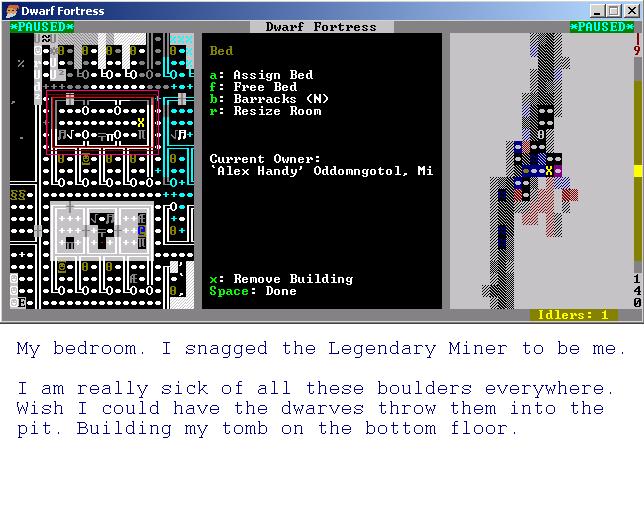This image is a detailed screenshot from the classic game "Dwarf Fortress," a text-based strategy and simulation game reminiscent of the 1980s-90s era of computer games. The game is paused, as indicated by green letters at the top center. The window's title bar at the top left reads "Dwarf Fortress," next to the minimize and close buttons, with a small dwarf icon nearby. On the right side of this bar, "Dwarf Fortress" is repeated. 

The screen features basic graphics, including a 2D image of a fortress-building, specifically a bedroom. In the middle section, there's a text-based interface with instructions and information. The interface details include options such as "A" for assigned bed, "F" for free bed, "B" for barracks, and "R" for resized room. It also displays the current owner’s name, Alex Hanby, and other contextual commands like "X" to remove building and "space" to finish the action.

Below the screenshot, white text on a blue background reads, "My bedroom. I snagged the legendary miner to be me. I'm really sick of all these boulders everywhere. I wish I could have the dwarfs throw them into the pit, building my tomb on the bottom floor." There's additional text on the left side of the screen, probably part of an interactive map typical for games of this genre, complementing a larger map on the right side.

The overall aesthetic and gameplay elements create an immersive Dungeons and Dragons-like experience, characteristic of early adventure and strategy computer games.